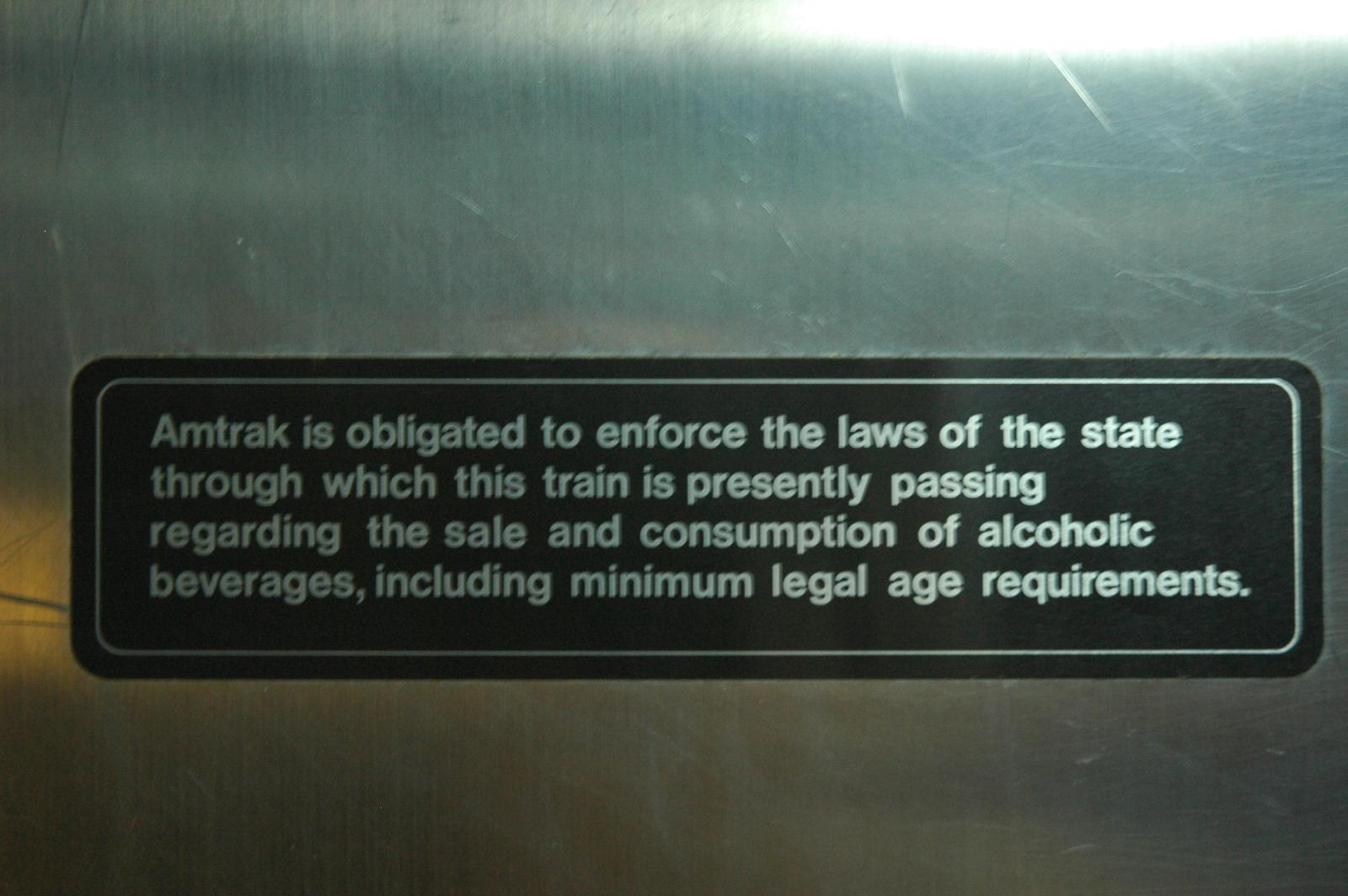The image depicts a cautionary sign in the form of a rounded rectangular plaque with a black background and a thin silver border. The sign features silver or white lettering that reads, "Amtrak is obligated to enforce the laws of the state through which this train is presently passing regarding the sale and consumption of alcoholic beverages, including minimum legal age restrictions." The period at the end of the statement is clearly visible. The plaque is affixed to a metal surface, likely stainless steel, which shows noticeable scratches. There's a bright reflection of light emanating from the top right corner of the sign, spreading nearly halfway across the surface. The background outside the frame of the sign looks like it might be rainy, with faint indications of drizzle.